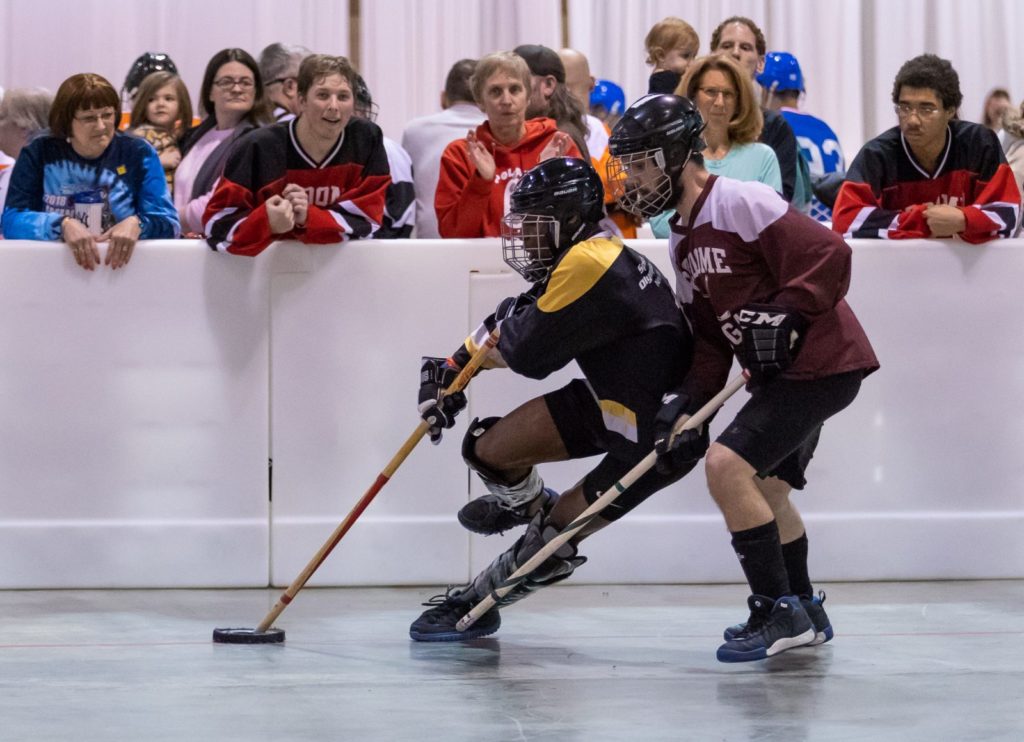In this clear and brightly-lit image, two players are engaged in a lively floor hockey match on a smooth gray surface. The player on the left, dressed in a black and yellow uniform, is in close contention with the player on the right, who sports a maroon, white, and black outfit. Both players are equipped with hockey helmets and gloves, and instead of skates, they wear regular shoes suitable for floor hockey. Their sticks are positioned towards the bottom left of the image, where the puck is located. Behind them stands a white barrier wall, beyond which are spectators bundled in winter attire, suggesting a cold environment. Among the diverse audience, a young girl being held by her mother and an older woman can be spotted. The background consists of additional white walls with draped coverings, completing the scene of this energetic and engaging sporting event.